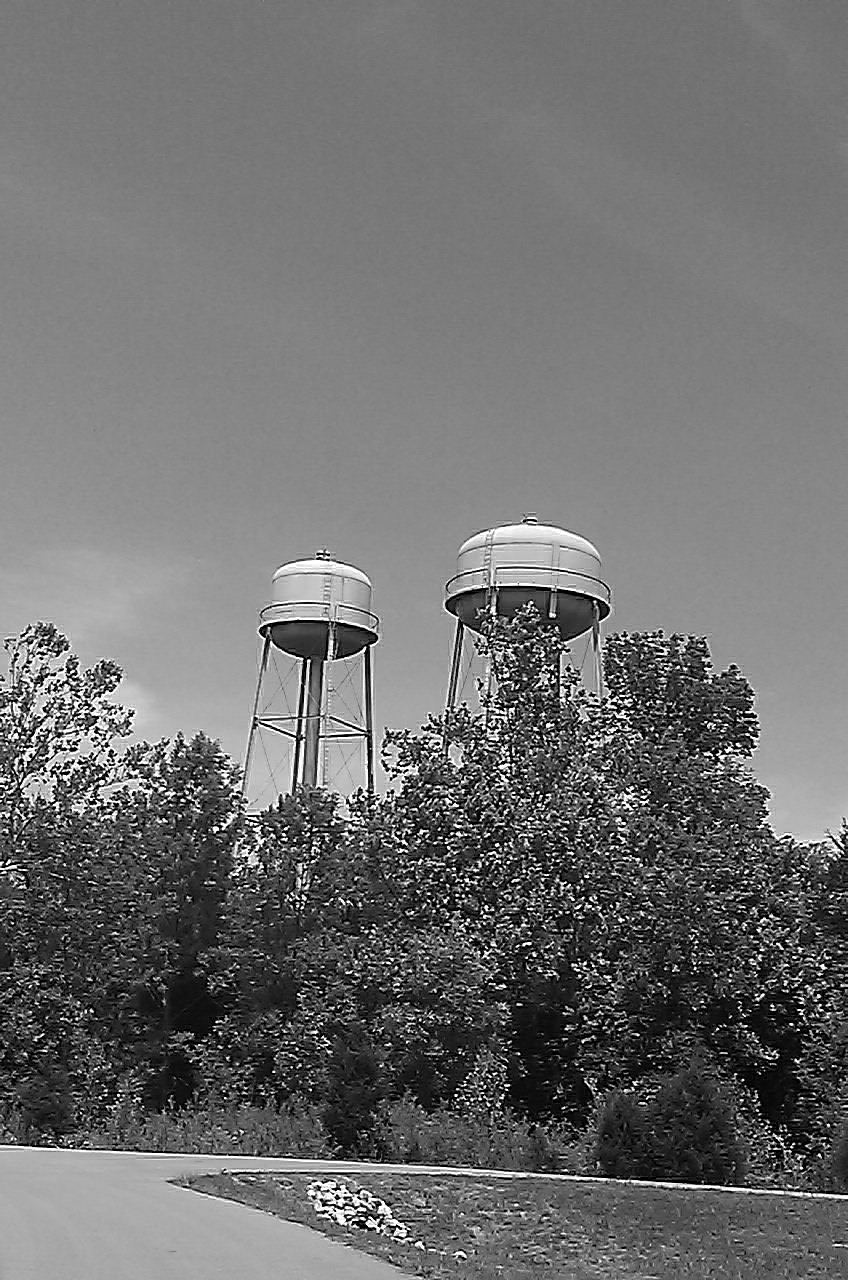This black-and-white photograph captures two water towers side-by-side, both elevated on a tall metal stand with steps leading up to each tank. These water towers, which lack any markings or letters, dominate the center of the image, with the larger and wider one slightly closer to the foreground and the smaller one set a bit further back to the left. In front of the water towers are tall, leafy trees, with some scrubby vegetation below them. Stretching across the bottom right corner of the image is a roadway or pathway that curves to the right, encircling a grassy area dotted with small rocks or large pieces of gravel. The sky above is a gradient of gray, appearing lighter due to the black-and-white nature of the photograph, suggesting a sunny and hazy day. The scene is devoid of people or animals, and the overall setting suggests a quiet, almost still environment.